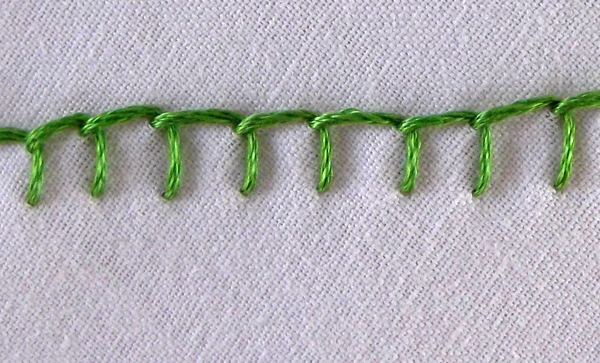This highly detailed close-up photograph captures a series of green threaded stitches embedded in a white fabric background. The fabric appears to be an off-white or grayish color, resembling either a well-woven cloth or a durable paper towel. Each stitch forms an open-ended square pattern as the thread weaves its way from the left to the right of the image, looping up and down across the material. This creates a slightly uneven, but consistent line of about eight or nine stitches. The green thread is shiny and medium in color, giving the impression of a forest of abstract trees when observed closely. The meticulous depiction reveals the texture of the fabric and the precise, albeit roughly executed, positioning of the stitches, set slightly above the center of the image.